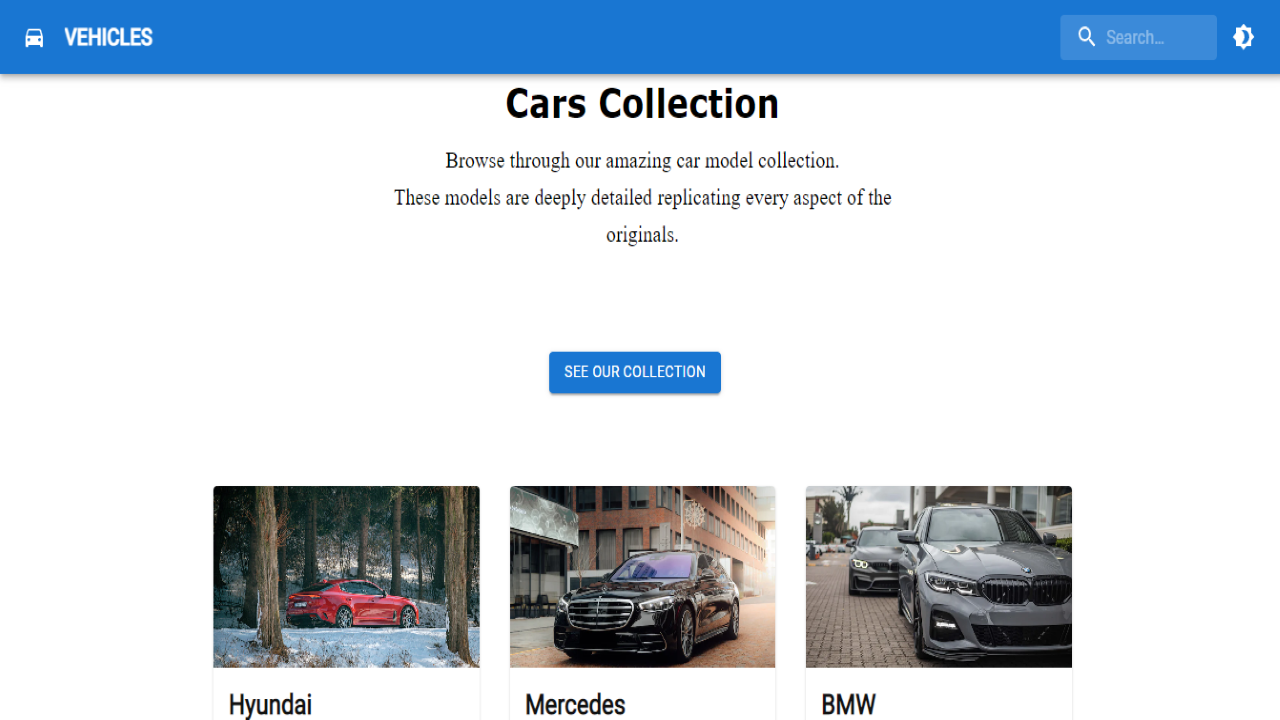This image is a screenshot of a car dealership website dedicated to selling vehicles. The webpage features a clean, organized layout with a blue header and a predominantly white background. In the top left-hand corner, there is a "Vehicles" button, accompanied by a small icon of a car to its right. On the opposite corner, the top right-hand side of the page, there is a small search bar followed by a contrast adjustment button depicted as an icon of the sun overlapping with the moon.

At the very top of the website, the heading "Cars Collection" is centrally placed, inviting users to "Browse through our amazing car model collection. These models are deeply detailed, replacing every aspect of the originals." Directly beneath this header, a prominent blue rectangle button labeled "CR Collection" offers easy navigation.

Below the button, the main content displays three car images side by side, each with the make of the car listed below. The leftmost image shows a red Hyundai car, the center image features a black Mercedes car, and the rightmost image displays a gray BMW car. The page maintains a simple aesthetic with a blue header offsetting the crisp white background, ensuring that the car images and essential information stand out to the viewer.